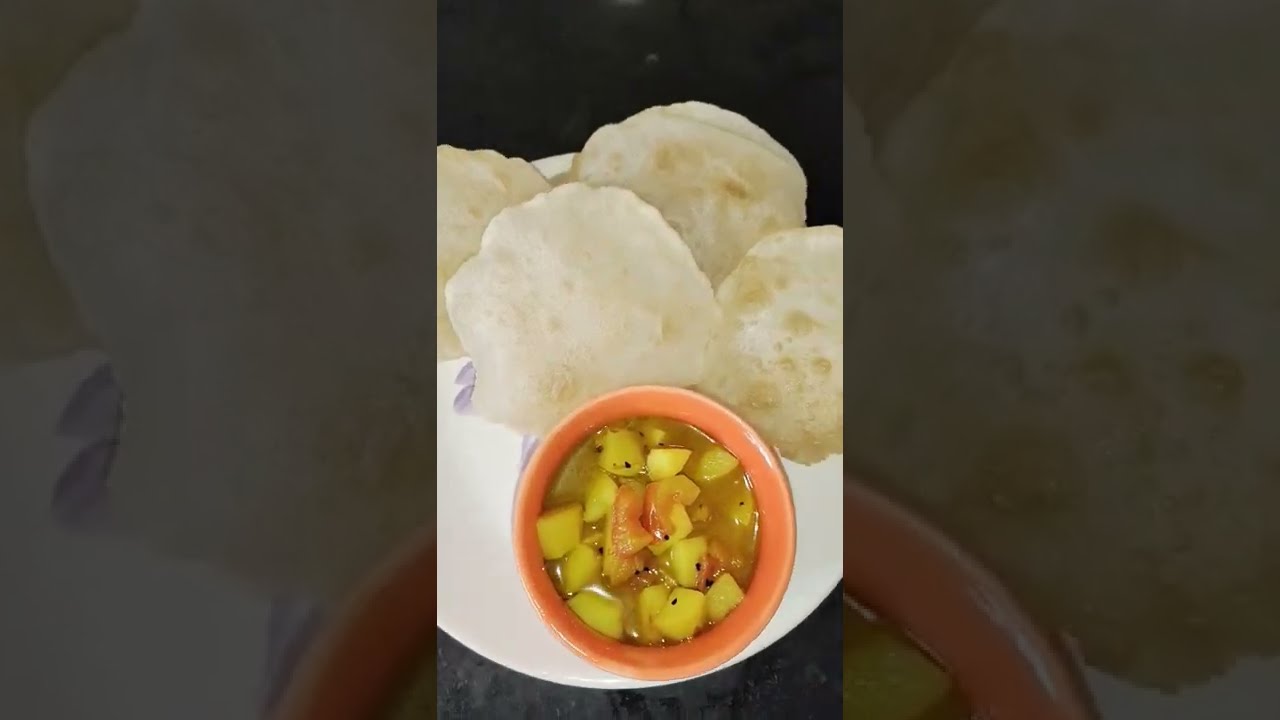The image captures an overhead view of a small meal set on a gray granite tabletop. A white plate with a subtle purple flower design hosts four light-colored homemade tortillas that resemble full moons with their distinct rounded, browned areas. Below the tortillas, there's a small orange bowl containing a pale-colored fruit sauce or condiment, featuring small cut-up yellow pieces—potentially a mix between pineapple and melon, speckled with black seeds. The entire composition is framed by a larger, darkened, and slightly zoomed-in version of the same image, creating a repetitive, layered effect where sections of the orange bowl and tortillas appear on both the left and right sides of the main photo. This intricate setup gives the meal a focal prominence against the minimalist, textured background.